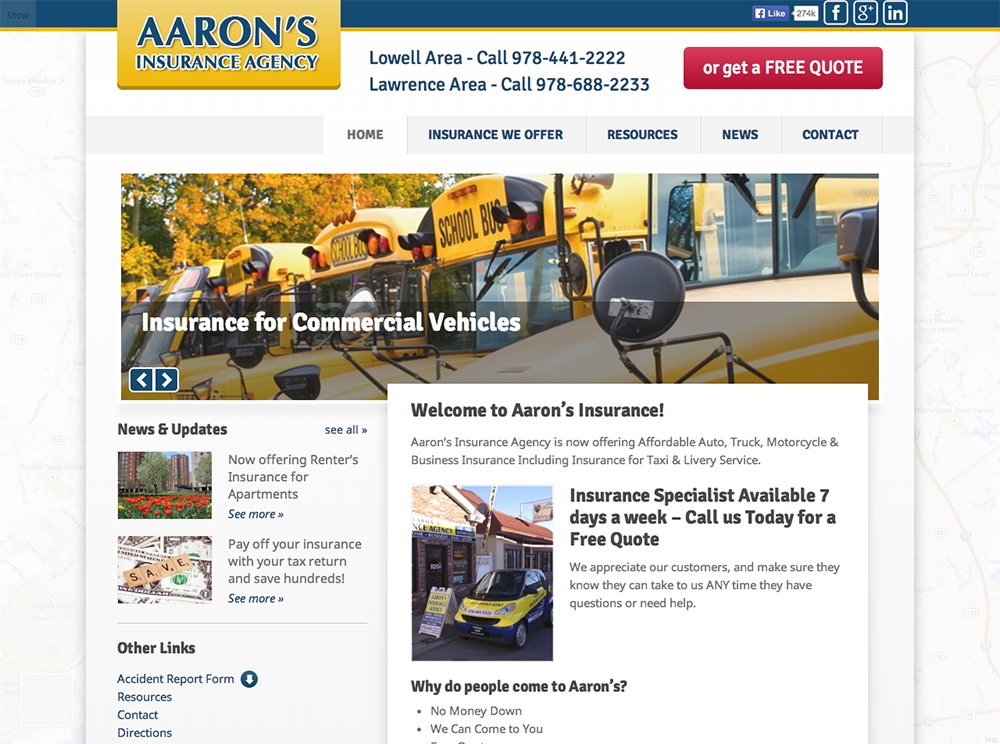### Detailed Caption:

The image appears to be a screenshot taken on a computer, showcasing the website of Aaron's Insurance Agency. The very top of the screen is marked by a distinct blue line. Just past the left edge of the screen, a visible yellow rectangle highlights the company's name, "Aaron's Insurance Agency," displayed prominently in blue letters.

In the upper right corner, there are social media icons, including a square labeled with an "F" for Facebook and another with a "G" for Google Plus. The website features a clean, white background. Centrally positioned at the top, the text provides contact information: "Lowell area call 978-441-2222" and "Lawrence area call 978-688-2233." To the right of this contact information, a conspicuous red rectangle invites visitors to "get a free quote."

Beneath this header, navigation options are listed: Home, Insurance We Offer, Resources, News, and Contact. Dominating the middle section of the page is a large image that spans the full width of the screen, depicting a row of yellow school buses. On the left side of this image, text reads "Insurance for commercial vehicles."

A pop-up screen is visible to the right, greeting visitors with "Welcome to Aaron's Insurance." The pop-up notifies readers that Aaron's Insurance Agency now offers affordable insurance options for autos, trucks, motorcycles, and businesses, including specialized insurance for taxi and livery services. It also highlights that insurance specialists are available seven days a week and encourages potential clients to call for a free quote.